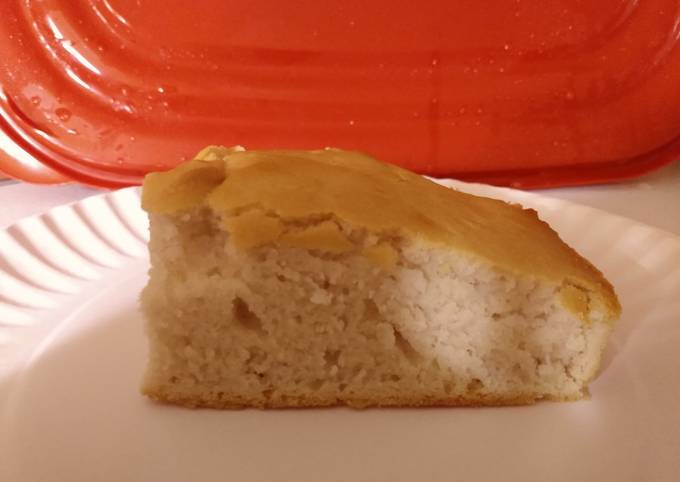This image showcases a small slice of homemade cake placed on a white paper plate with traditional ridged edges. The cake features a light golden brown crust on both the top and bottom, while the interior is a dense, thicker, off-white center dotted with tiny air pockets, indicating a soft texture. Positioned on a white counter, the plate is set in front of a wet, red Tupperware lid with a rounded edge and a small extension used for snapping it into place. The close-up view emphasizes the cake's homemade quality and the details of the crimped paper plate and the intricate design of the lid in the background.